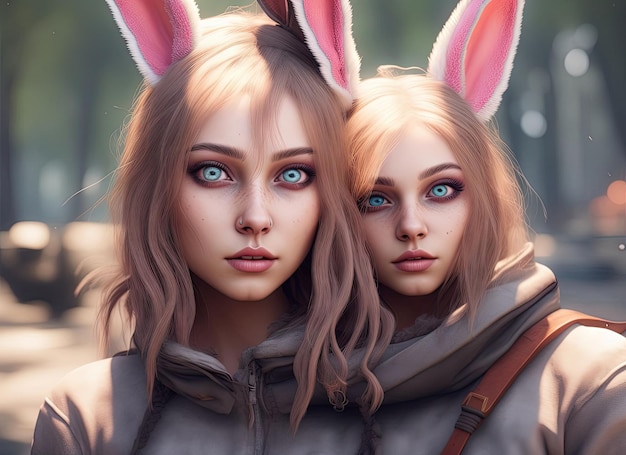This AI-generated image from The Look of Things portrays a pair of teenage girls who overwhelmingly resemble each other, possibly suggesting they are sisters. Their striking electric turquoise eyes, emphasized by artfully applied eyeshadow and eyeliner, dominate the image. Both girls have flowing strawberry blonde hair that frames their youthful faces. Each wears pink bunny ears with white fur lining the outer edges. They are dressed in gray sweaters that appear to have hoods, although one of the girls also has a tan leather strap over her left shoulder, likely for a purse. The girls' light makeup complements their natural beauty, featuring very pink lips and distinct eyebrows. The background is a blur, eliminating any discernible details of their surroundings and keeping the focus solely on the girls. The anime-style art suggests a blend of natural and surreal elements, as their vibrant eyes and seamlessly combined shoulders give the impression of a whimsical, almost fantasy-like scene. Despite their symmetrical features and connected appearance, subtle differences such as height distinguish one from the other.